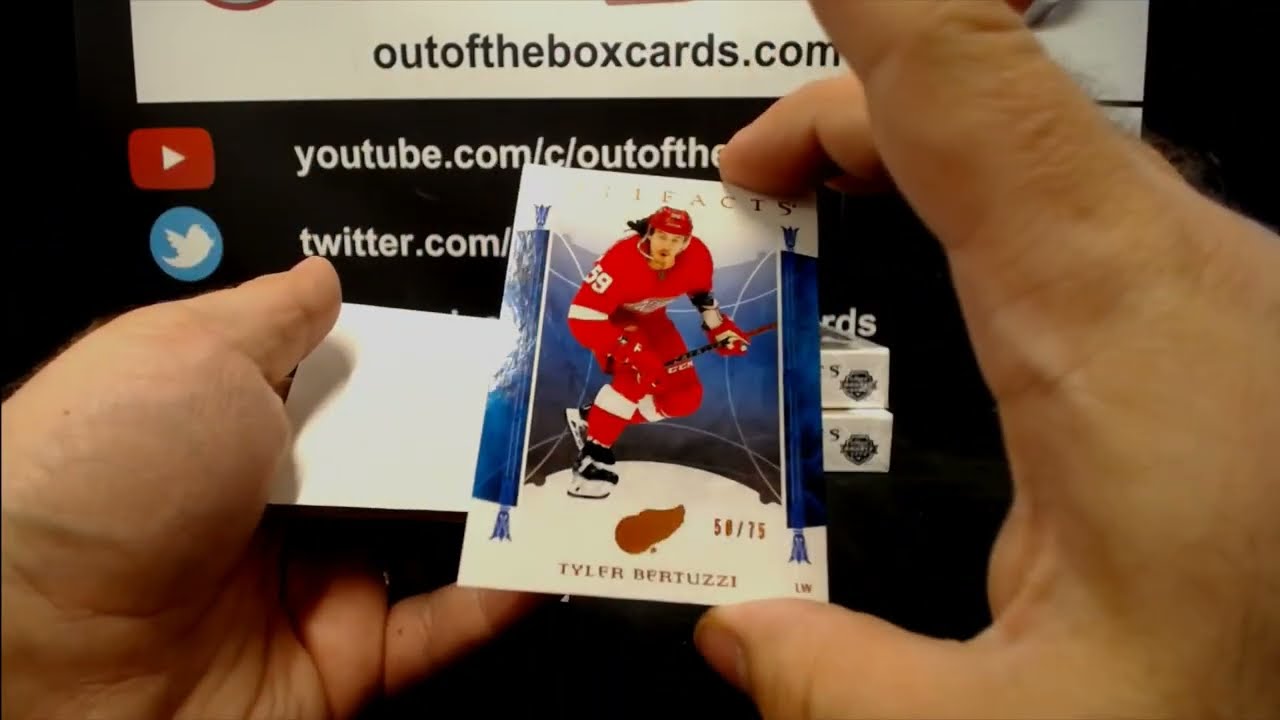The photograph depicts a close-up of a man's hands holding a hockey card with an air of reverence. The card, predominantly white, features an image of Tyler Bertuzzi in a red uniform with white stripes and a red helmet, poised with a hockey stick. Bertuzzi has long hair and the number 59 is visible on his shoulder. The name "Tyler Bertuzzi" is printed at the bottom of the card in black-brown text. 

In the background, a tablet is held in the man's left hand, displaying a website with the heading "out-of-the-boxcards.com" in black text. Below that, additional text includes "youtube.com/out-of-the-box cards" and "twitter.com," though parts of the URLs are partially obscured. The remainder of the background is black, highlighting the card and the tablet. The scene is well-lit, with a bright light source illuminating the top left corner and left edge of the card, accentuating the details of the player's image and the card's text.